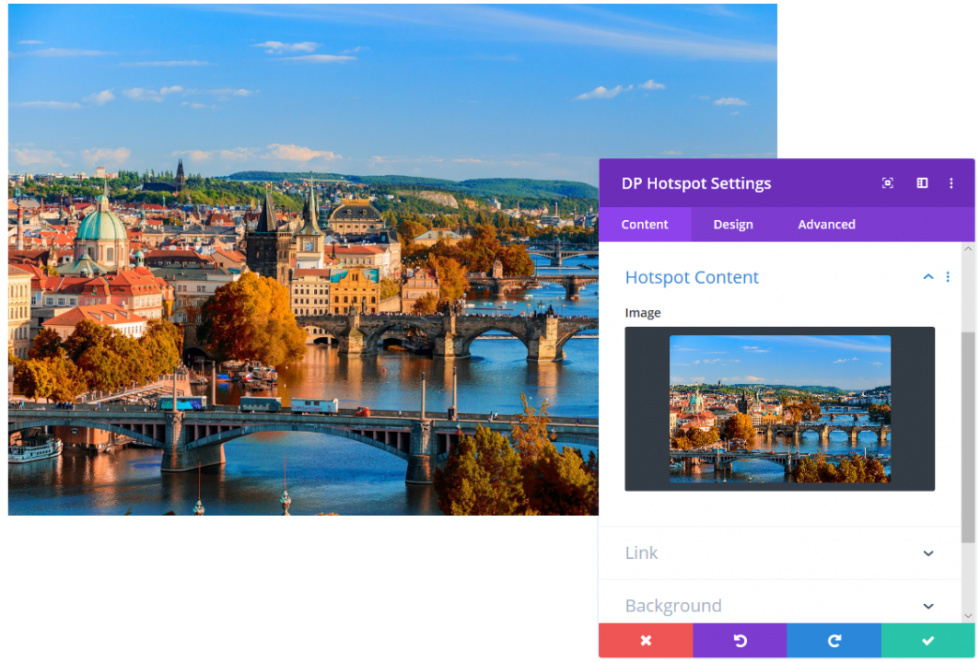This captivating image showcases a picturesque scene of a beautiful location, featuring multiple gray stone bridges gracefully spanning a large, dark blue river. To the right, a pop-up window is visible, suggesting image editing features with tabs labeled: "Hotspot Content," "Settings," "Hotspot," "DP Hotspot Settings," "Content Button," "Design Button," and "Advanced Button." Additional buttons include a "Link Tab," a "Drop-down Button," and a "Background Button." 

Focusing back on the main photograph, to the left of the bridges and river, there is a cluster of buildings with striking orange roofs surrounded by lush, light green trees. In the foreground, there is what appears to be a truck or train crossing the nearest bridge. Dominating the background are large, rolling, dark green hills that add depth to the scene. 

At the bottom right of the editing pop-up, several control buttons are neatly arranged: an "X" button for exiting, a back button, a forward button, and a checkmark button for confirming selections. This detailed composition offers not only a breathtaking view of the location but also an insight into the digital tools used to enhance and manage visual content.